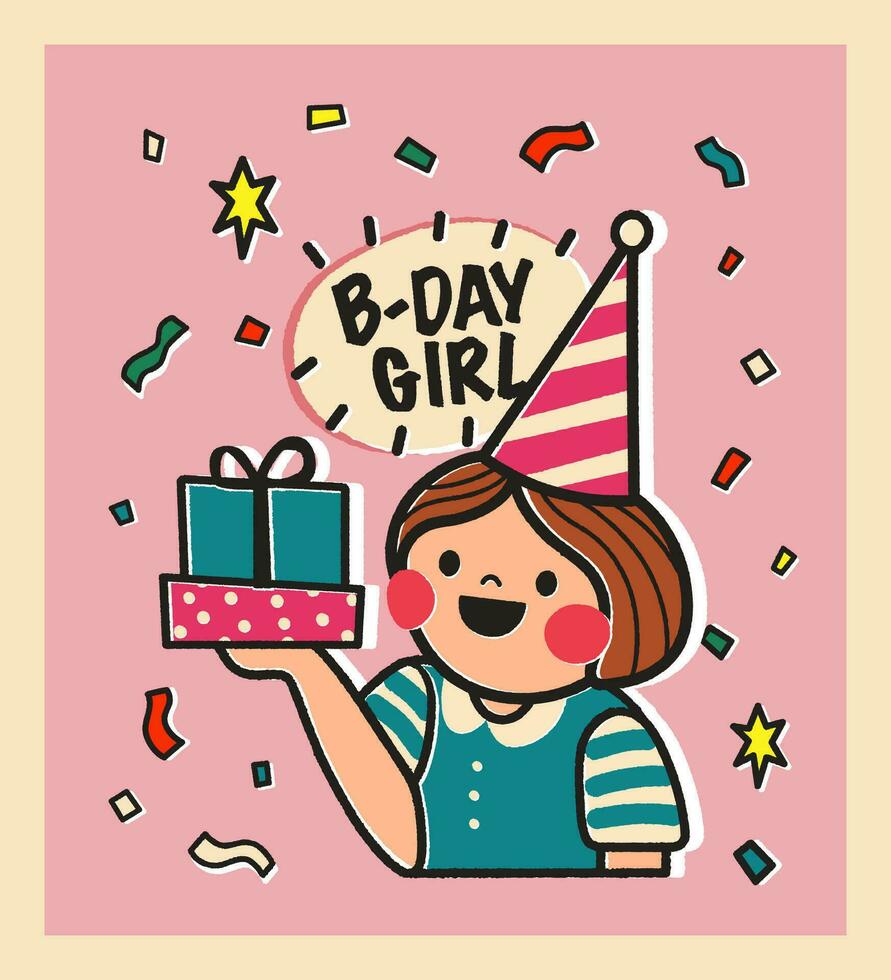The image is a vertically rectangular, multi-colored print piece with a light brown (ivory) border and a pink background adorned with stars and confetti in various colors including pink, yellow, green, white, and red. At the center of the image is a hand-drawn or digitally created illustration of a little girl with brown shoulder-length hair and two red circles for rosy cheeks. She is wearing a short-sleeved blue and white striped shirt and a red and white striped party hat with a white ball at the top. Above her head, the text "B-Day Girl" is prominently displayed. The girl holds two wrapped presents in her hands, one pink and one blue, symbolizing a festive birthday celebration. She is facing towards the left with her right hand raised, adding to the scene's lively atmosphere.